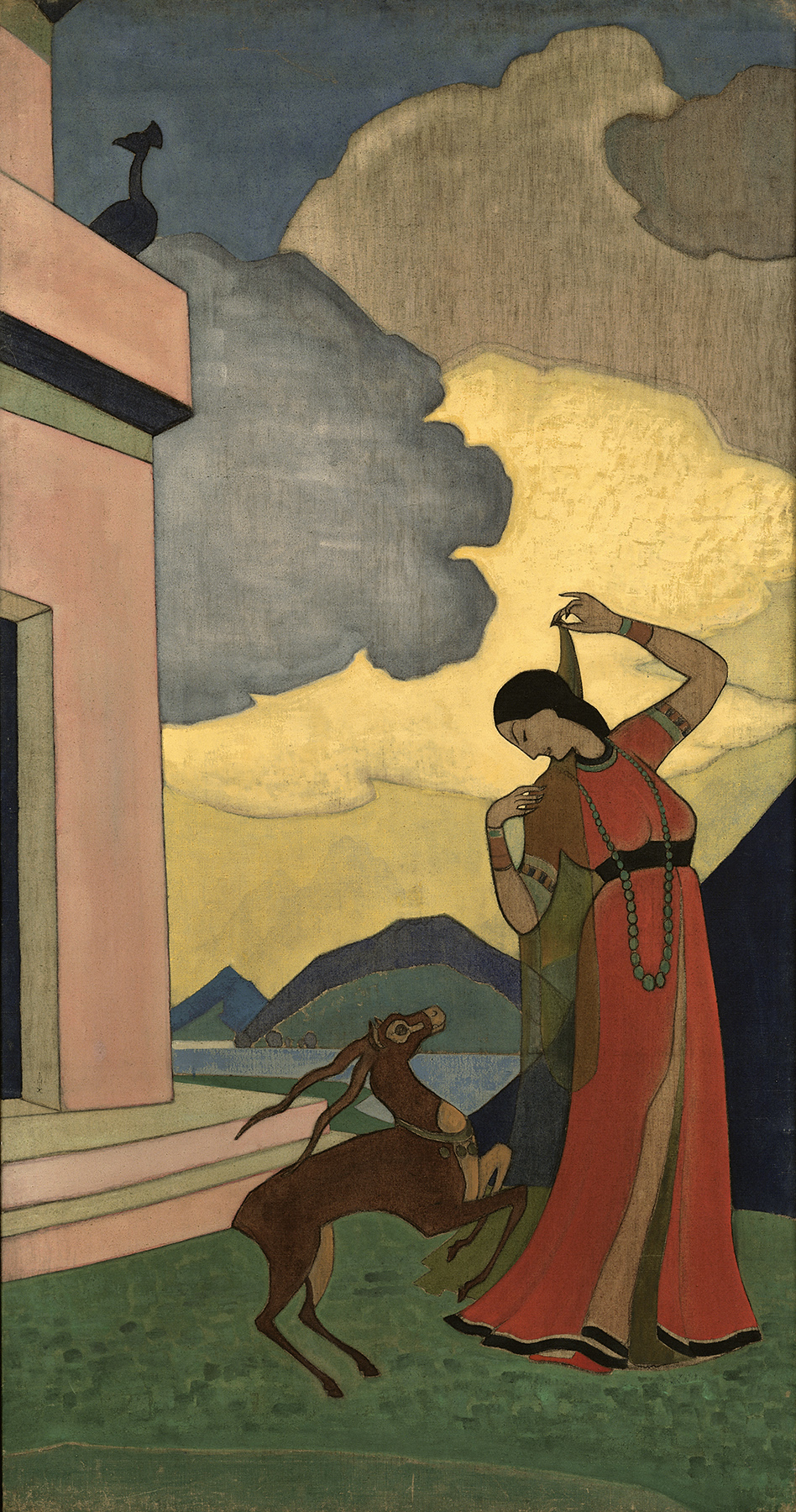This vertically aligned rectangular painting features an evocative sky at the top, dominated by a blend of dark gray and blue hues. Interspersed within the sky are clouds of brown, yellow, gray, and white, arranged with irregular, curved borders. The left side of the painting depicts a pink-hued structure, possibly an ancient temple or modern building, with a black-shaded stork or long-necked bird perched on its roof. Two pink stairs with gray tops descend from a partial doorway visible on the far left.

In the foreground, a woman stands on the grass to the right side. She wears a flowing red gown paired with a long, beaded necklace that extends well past her waist, and a black belt around her waist. A sheer, brownish lace shawl is draped over her shoulders, held up by her raised left arm. She has long black hair and is adorned with bracelets on both wrists. Her head is tilted downward with closed eyes, gazing upon a small animal on its hind legs—a creature resembling a deer or antelope with tiny horns, poised as if about to leap towards her. The background of the painting hints at rolling hills and possibly a distant body of water, merging the elements of antiquity and modernity through stylized, almost caricatured clouds.